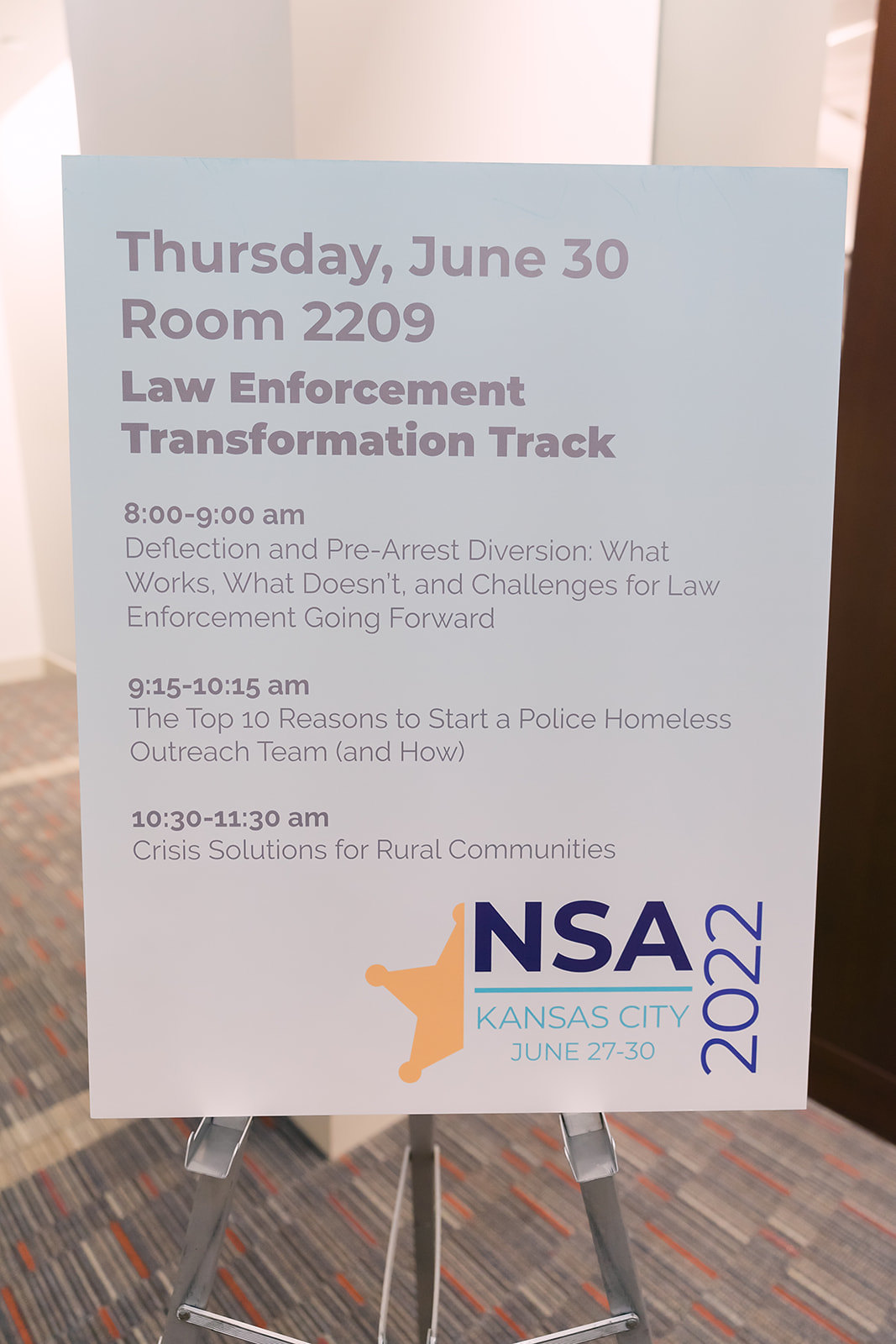The photograph depicts a poster on a metal stand advertising a seminar series. The poster has a white background with multiple lines of black text. At the top, in large letters, it reads, "Thursday, June 30." Directly below, it indicates the location: "Room 2209," followed by the title "Law Enforcement Transformation Track" in slightly smaller but still prominent typography. 

The seminar schedule is detailed in three sections with specific times and topics:
- From 8 to 9 a.m., the session titled "Deflection and Pre-Arrest Diversion: What Works, What Doesn't, and Challenges for Law Enforcement Going Forward."
- From 9.15 to 10.15 a.m., a session on "The Top Ten Reasons to Start a Police Homeless Outreach Team (and How)."
- From 10.30 to 11.30 a.m., a session on "Crisis Solutions for Rural Communities."

In the bottom right corner of the poster, there is an insignia featuring half of a gold sheriff's star and the text "NSA" in bold letters with a light blue underline. Below "NSA," it reads "Kansas City" in light blue all caps, and "June 27 to 30." Vertically aligned alongside, the year "2022" is displayed. The background scene includes gray carpet with orange and cream stripes and illuminated white walls.